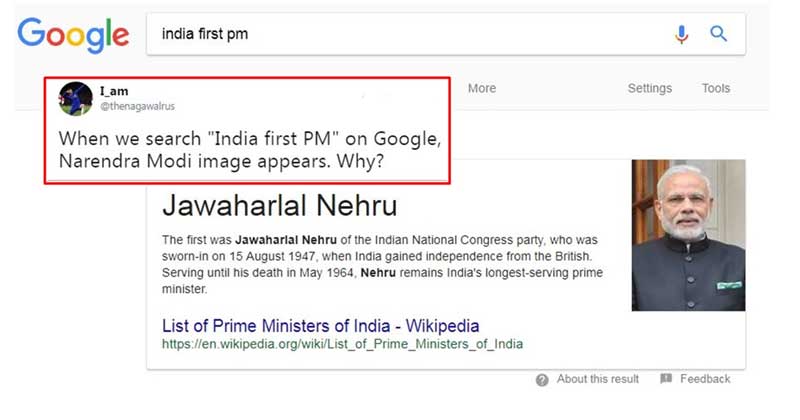The image in question depicts a detailed interaction regarding the inquiry of India's first Prime Minister on Google. On the left, there's the recognizable Google logo, adjacent to a search box featuring a microphone icon beside the standard magnifying glass.

At the center of the image is a tweet from the user @imthenagawal, expressing confusion over the search results for "India 1st PM." The tweet specifically reads: "When we search India 1st PM on Google. Not Narendra Modi appears, why?"

Below the tweet, the Google search results are displayed, correctly indicating Jawaharlal Nehru as India's first Prime Minister. The search result snippet provides a brief overview:

"Jawaharlal Nehru, the inaugural Prime Minister of India, was sworn in on August 15, 1947, following the nation's independence from British rule. He remained in office until his death in May 1964, making him the longest-serving Prime Minister of India."

This is followed by a link to a Wikipedia article titled "List of Prime Ministers of India."

On the right, the address bar of the search page is visible, along with an image of an elderly Indian man dressed in a military-style jacket, presumed to be Jawaharlal Nehru. This image, however, has led to the user's confusion, as they mistakenly associated the query with Narendra Modi, the current Prime Minister of India.

Overall, the image encapsulates the user's bewilderment at the accurate yet unexpected search result regarding India's first Prime Minister, emphasizing common misconceptions about historical figures among the general public.